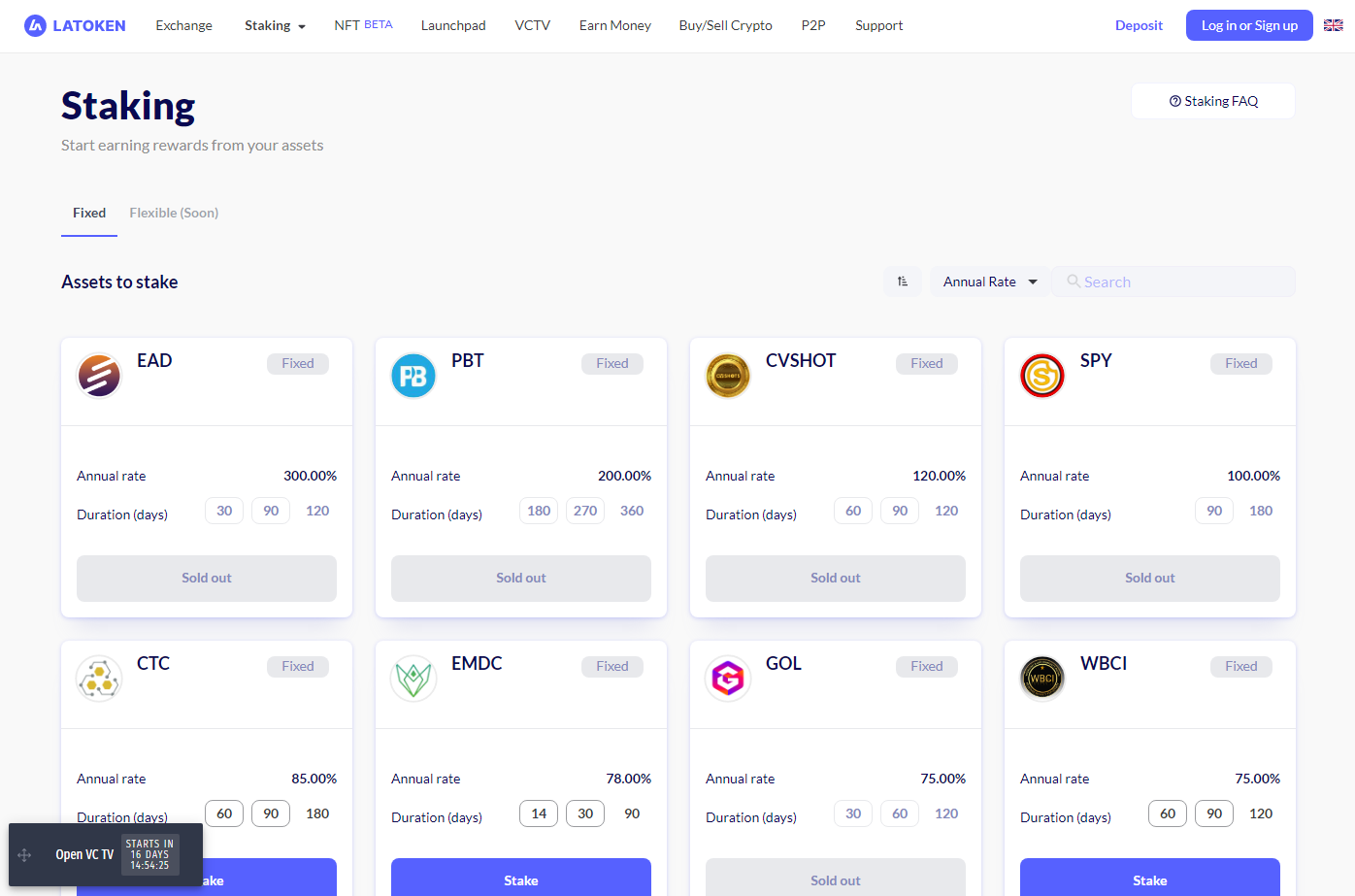**Detailed Descriptive Caption:**

The image showcases a detailed overview of various cryptocurrency investment options on a trading platform. At the top of the list, prominent features like "Token Exchange," "Net Beta," "Dodgepad," and "PCTV" are emphasized for their capability to help users earn money through buying and selling cryptocurrencies. The platform supports P2P transactions, with a focus on deposits, highlighted with a blue rectangular banner.

Additionally, there's a clear call to action for users to log in or sign up, depicted with a registration flag icon. The platform offers staking opportunities, where users can start earning rewards on their assets through programs like "Tickify" which offer both fixed and flexible sums, coupled with detailed asset statistics. Annual rates and various durations for investment options are meticulously displayed with corresponding icons.

There are numerous investment plans, each labeled with specifications. For instance, "AAD" offers fixed annual rates of 300% for durations of 30, 90, and 120 days, although these options are marked as sold out. Other plans such as "DBT" provide annual rates of 200% for durations of 180, 230, and 360 days, also sold out. Under the "CB Shot" category, multiple durations like 60, 90, 120, 180, and 230 days at an annual rate of 120% are all marked sold out.

Towards the end, the image indicates the final results of an offering called "OpenVC2," which is set to start in 16 days from the date referenced, specifically marking 14.4.25 as the subsequent date. This comprehensive layout is aimed at helping users to understand and engage with multiple cryptocurrency investment opportunities on the platform.